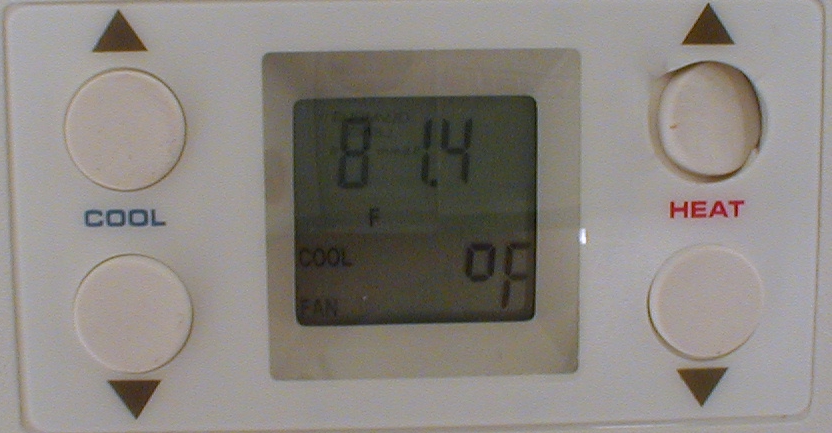This detailed photograph showcases a modern thermostat with a zoomed-in focus on its front panel, which is sleek and white with curved edges. The rectangular device, longer in width than in height, features two circular white buttons on its left side. Above the top button is a small brown triangle pointing upwards, and below the bottom button is a similar triangle pointing downwards. Between these buttons, the word "COOL" is printed in blue text.

On the right side of the thermostat, there are two additional buttons; the top one is fully pressed. Situated between these two buttons is the word "HEAT" in red text. Centrally positioned on the device is a digital screen with squared yet rounded edges. The screen displays "81.4°F COOL FAN" in a classic digital clock font, with "°F" appearing in the bottom right corner. The background of the display screen is a subdued greenish-gray, which contrasts well with the white exterior of the thermostat.